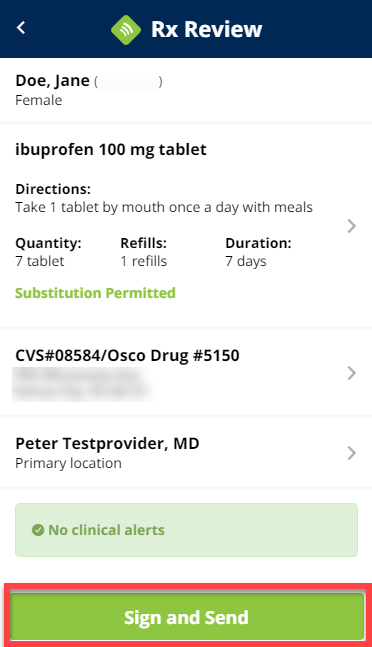**Detailed Caption:**

This screenshot displays a mobile app interface related to prescription information. At the very top, there is a dark blue, almost black, banner with a white left arrow on the left side, followed by a green box containing an icon of three wavy lines. Adjacent to the icon, the text "RxReview" is written in white letters.

Beneath the banner, the person’s details are presented on a white background: the name "Doe, Jane" in black text, and the gender "female." Below this, a gray line separates the personal details from the medication information.

The medication details follow: "Ibuprofen, 100 milligram tablet" in black text with smaller instructions below: "Directions: Take one tablet by mouth once a day with meals." Further details include: "Quantity: 7 tablets," "Refills: 1 refill," "Duration: 7 days," and in bold green text, "Substitution permitted."

Another gray line demarcates this section from the labeling information: "CVS number 08584," "Osco drug number 5150." There is a blurred text section with an arrow indicating a clickable link.

Further below, the provider information is displayed: "Peter Test, Provider, MD," and "Primary location," both of which are clickable links. 

Towards the bottom, a light green box displays a message in darker green text: "No clinical alerts," accompanied by a green check mark.

Finally, there is a green box with white text, outlined in a red border, that states: "Sign and send."